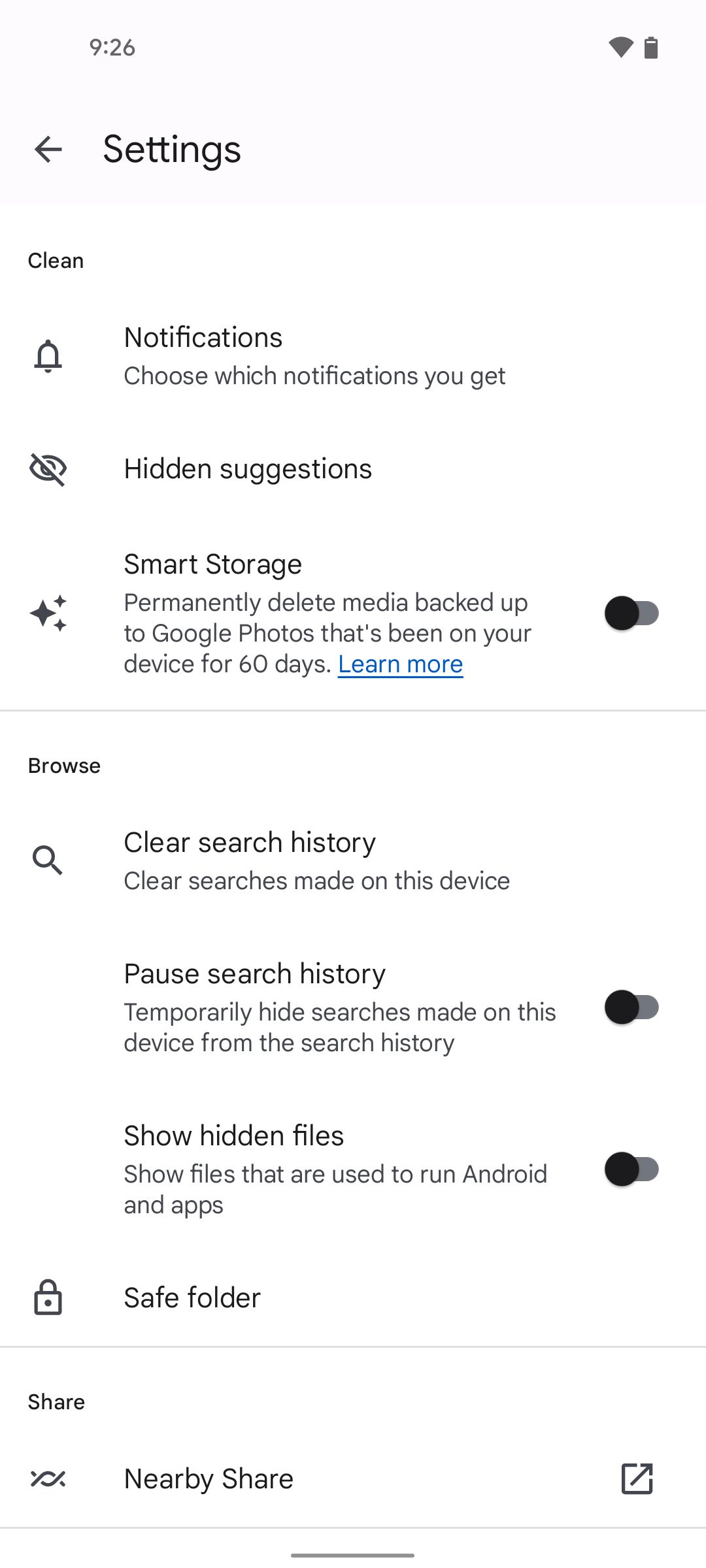The image depicts a settings menu on a mobile device. At the top of the screen, there is a gray background displaying the time "9:26" in the upper left-hand corner. On the right side, there are icons for full Wi-Fi connectivity and a battery at three-quarters capacity. Below this, a black back arrow pointing to the left is positioned next to the word "Settings".

The rest of the screen has a predominantly white background, displaying various menu options with icons and descriptions. The options are as follows:

1. **Clean**: 
   - **Notifications**: Choose which notifications you receive, represented by a bell icon.
   - **Hidden Suggestions**: Manage hidden suggestions, depicted by an eyeball icon with a cross through it.

2. **Smart Storage**:
   - Automatically and permanently delete media that has been backed up to Google Photos after 60 days. This option includes a "Learn more" link and is currently toggled off.

3. **Browse**:
   - **Clear Your Search History**: Remove searches made on this device.
   - **Pause Search History**: Temporarily hide searches made on this device from the search history, currently toggled off.

4. **Show Hidden Files**:
   - Display files that are used to run the Android system or apps, currently toggled off.

5. **Safe Folder**:
   - A secure area, indicated by a lock icon.

6. **Share**:
   - **Nearby Share**: Features an icon that looks like a crossed thread, enabling sharing with nearby devices.

This detailed layout of the settings menu provides a comprehensive overview of the various options available for managing notifications, storage, browsing history, and file visibility on the device.